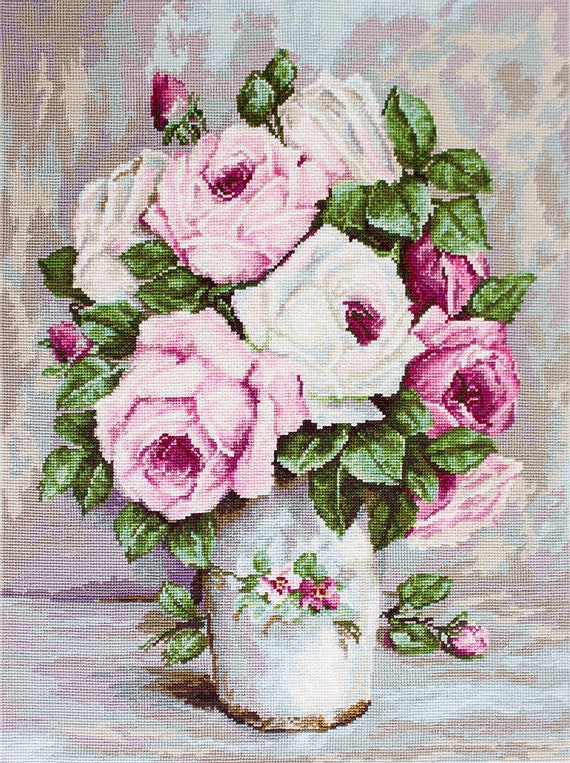This detailed needlepoint artwork showcases a stunning bouquet of roses in a white, gold-trimmed vase. The bouquet consists of blooming roses in varying shades of pink—from light to dark—with some featuring red centers, interspersed with lush green leaves. Complementing the main bouquet in the vase are a few delicate rosebuds at the top, and a full rose lying on the table, still attached to its green stem that curls around the vase. The background is a rich tapestry of colors including shades of blue, pink, beige, brown, gray, and purple, adding depth and contrast to the detailed floral arrangement. The surface on which the vase stands mirrors these hues, enhancing the textured, almost pixelated effect of the needlepoint craftsmanship.